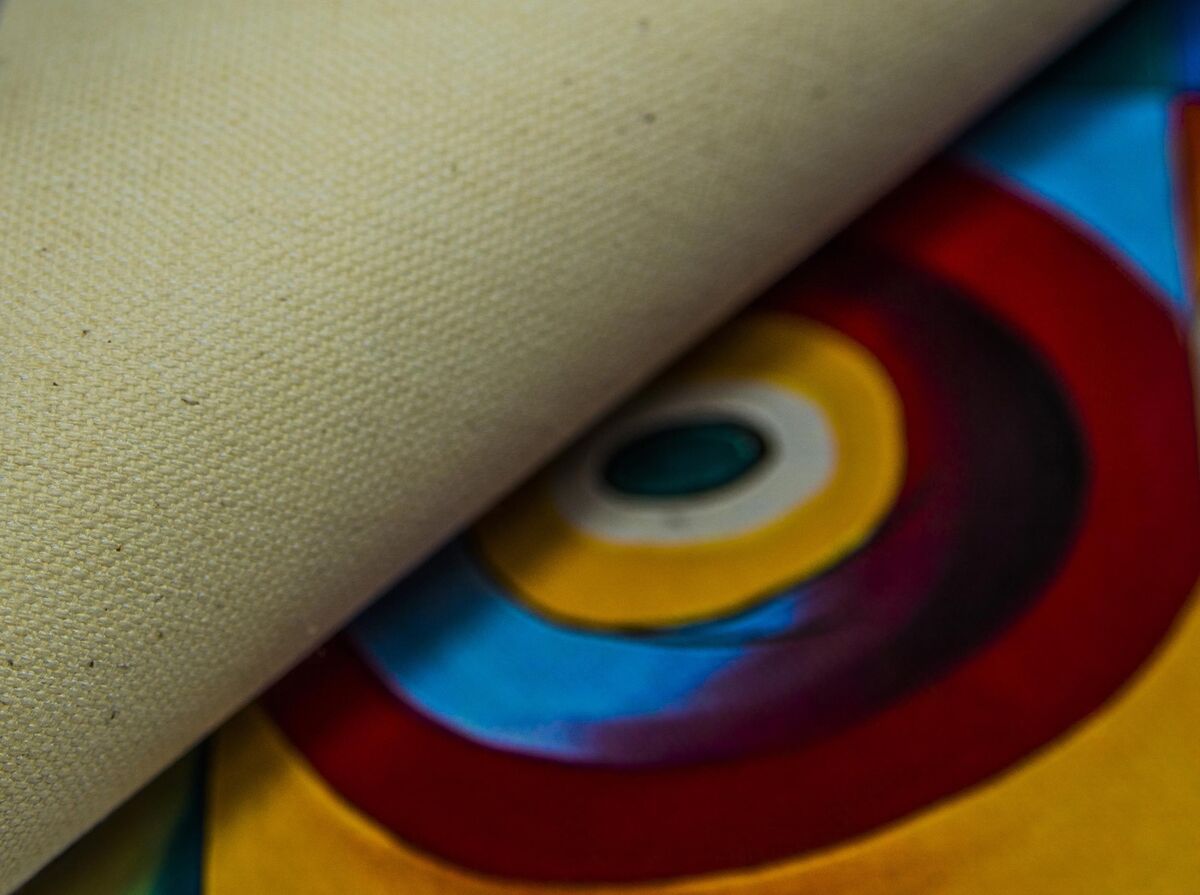This is an up-close photograph showing an intricate scene where a piece of white linen-like textile is half-folded over, covering the bottom left corner and tapering off diagonally towards the upper right corner, resembling a rolled-up carpet or placemat. This textile hides a circular, abstract design beneath that starts with a black central circle surrounded by concentric rings in varying colors: a white ring, followed by a yellow ring, a darker red and light blue segment, another red ring mixed with monochromatic shades of black to red, and an outer yellow section. The uncovered portion of the artwork dominates the bottom right corner of the image, lending a vivid contrast with its pop of multiple hues. The image, which seems to be either part of a book cover, piece of art, or album cover, measures approximately nine inches in width and seven inches in height and is rendered in medium quality without any accompanying text or visible people.